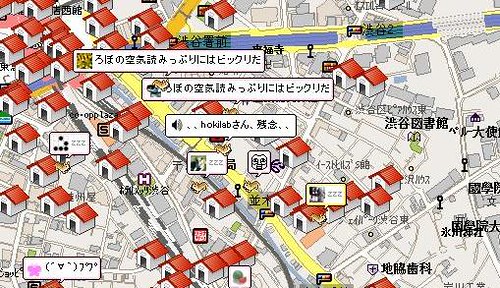The image is a detailed, color graphical illustration in landscape orientation, reminiscent of a freeze-frame from a video game. The scene depicts a bird's eye view of a populated neighborhood, complete with roads, train tracks, and waterways. Dominating the map are white, three-dimensional house structures with red pitched roofs, uniformly distributed along the grey-outlined streets. These houses feature large doors and are grouped, suggesting a gaming environment rather than an actual navigational map.

Text labels, predominantly in Japanese characters, populate the map and are enclosed in horizontally aligned rectangular boxes with thin pencil-style outlines. Some of these boxes contain "ZZZZ," indicative of sleeping figures, reinforcing the gaming context. Additional speech bubbles and possible animal figures, which appear to be bunnies or dogs, contribute to the whimsical, game-like atmosphere.

The map features a prominent yellow main road and a river or canal that meanders horizontally across the upper portion of the image. The map also shows various shades of grey to denote buildings and land zones, with minimal green areas, adding to the urban feel. Despite some pixelation, the intricate details evoke a vivid, immersive gaming level, complete with elements such as different colored roads and tram lines, enhancing the richness of the illustrated environment.